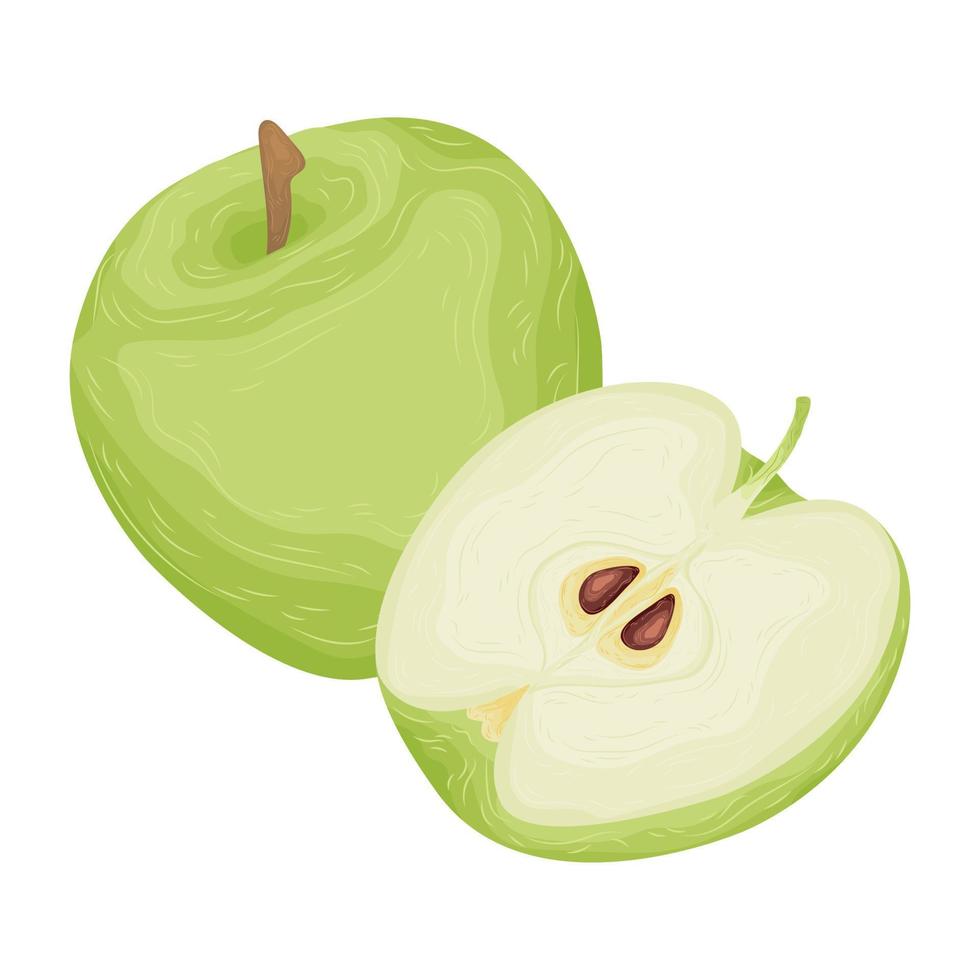This detailed illustration depicts a green apple and a cut half of a green apple against a white background. The whole apple resembles a Granny Smith variety with a smooth, vibrant green exterior painted in three different shades of green, along with white lines to add dimension and realism. It features a brown stem that starts narrow and becomes slightly larger towards the top. The cut half of the apple, positioned in front of the whole apple, reveals a light beige interior with two brown seeds clearly visible. Unlike the whole apple, the core and stem of the halved apple are entirely green without any brown. The interior of the halved apple also includes outlines of the apple's natural structure, enhancing the depth and texture of the painting.